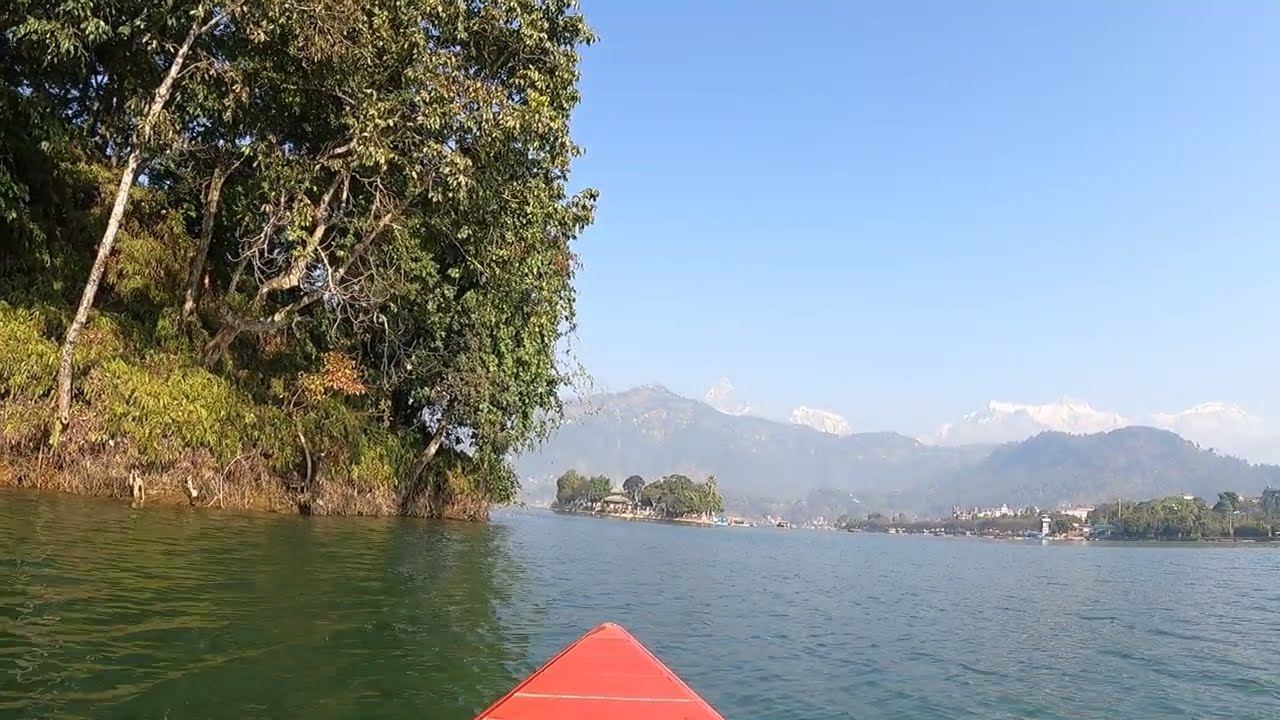The photograph, taken from the perspective of a person in a red kayak or canoe, showcases a breathtaking outdoor landscape. The kayak's bright orange or red tip is visible at the bottom center of the image, confirming the point-of-view angle of the shot. The vessel is floating on a large, greenish-blue body of water, possibly a lake. On the left side of the image, there is close land characterized by lush green grass, trees, shrubbery, and tall sides with roots visibly growing out. Further back on the left, the terrain appears to be a muddy hill that drops directly into the water.

In the middle and right sections of the image, majestic mountains rise into the light blue sky. Some of these peaks are capped with snow, while others are covered in green vegetation. Low-hanging clouds can be seen caressing the mountain peaks, although the main expanse of the sky is clear. 

To the right, in the distance, there appears to be a small village or a water-adjacent city nestled among more trees, adding a touch of human presence to the otherwise natural scene. The palette of the photo includes a variety of colors: brown, black, white, gray, green, yellow, pink, and multiple shades of blue. There are no visible living creatures, making the image a pure representation of the serene and unspoiled outdoors.